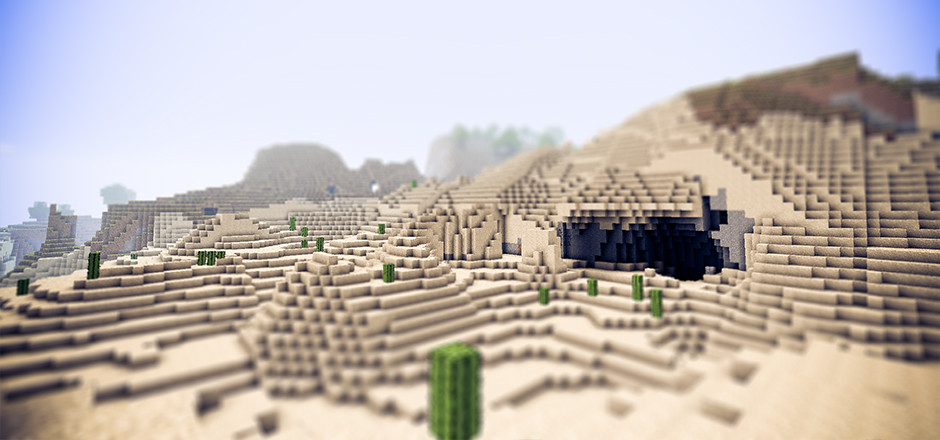The image appears to be a screenshot from Minecraft, showcasing a pixelated, desert-like landscape that resembles a scene from a computer or AI-generated world. The terrain is composed of blocky, tan and beige structures that somewhat mimic pyramids, with various mounds and terraces giving it a rugged, uneven appearance. Scattered throughout the scene are small, green, cube-like formations that could represent cacti or bushes. This composition creates an impression of ancient ruins or a desert with hills, with the right-hand corner of the image featuring darker shades of brown and gray, adding depth and contrast to the scene.